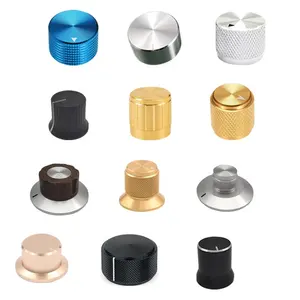The image showcases a meticulously arranged set of 12 knobs, organized into three rows with four columns each, all set against a clean white background, giving a clear and unobstructed view of every detail. The knobs exhibit a variety of colors, shapes, sizes, and textures, demonstrating a diverse collection.

In the top row, the first knob is a royal blue metallic with a textured outer rim and a smooth top marked by a small white triangle. The second knob is silver and identical in design to the blue one. The third knob in this row is another silver variant, resembling the first two.

The second row starts with a black knob featuring a white line that travels across its top and down its side. The middle knob is gold with vertical lines descending its sides, while the final knob in this row mimics the blue and silver design with a gold finish and textured sides, capped with a small white triangle.

The third row begins with a knob that has a white-silver core, surrounded by black and ending in a saucer-like bottom adorned with a short black line. Next, a gold knob with textured sides and a smooth top extends into a similar saucer-like base. The final item in the row is a silver knob characterized by a smaller, raised knob design atop its saucer-like base.

In the final row, a rose gold-colored knob has a slightly flared bottom edge, followed by a straightforward black knob marked with a white line down its side. The last in this row is a thinner black knob with a silver ring at the top and a white dash on its surface.

The collection displays a range of designs from simple cylindrical shapes to more complex forms with rounded bottoms, textured grips, and various accents, meticulously presented like a catalog of ornate appliance knobs.